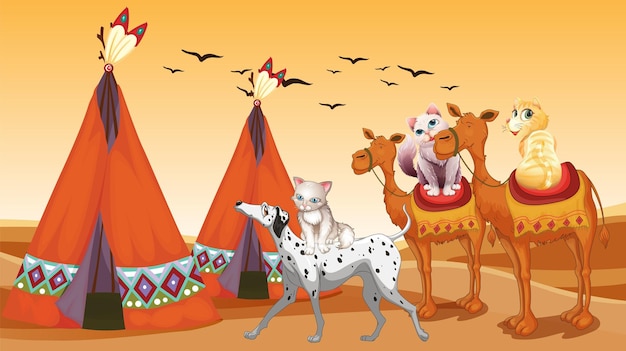This vibrant cartoon illustration depicts a whimsical desert scene, reminiscent of a children's book. Dominated by shades of brown and deep orange, the setting features two teepee-style structures with colorful tribal patterns near their bases and topped with eagle feathers. The scene includes charming, cartoon-proportioned animals: two smiling camels stand to the right, each ridden by a uniquely colored cat—one yellow, glancing over its shoulder, and the other purplish-white, looking upward. In front of the camels, a Dalmatian dog strolls with a gray cat perched on its back. Birds soar in the yellow-tinged sky, suggesting a sunset. The overall image, likely digitally rendered, exudes a playful and engaging atmosphere ideal for young audiences.